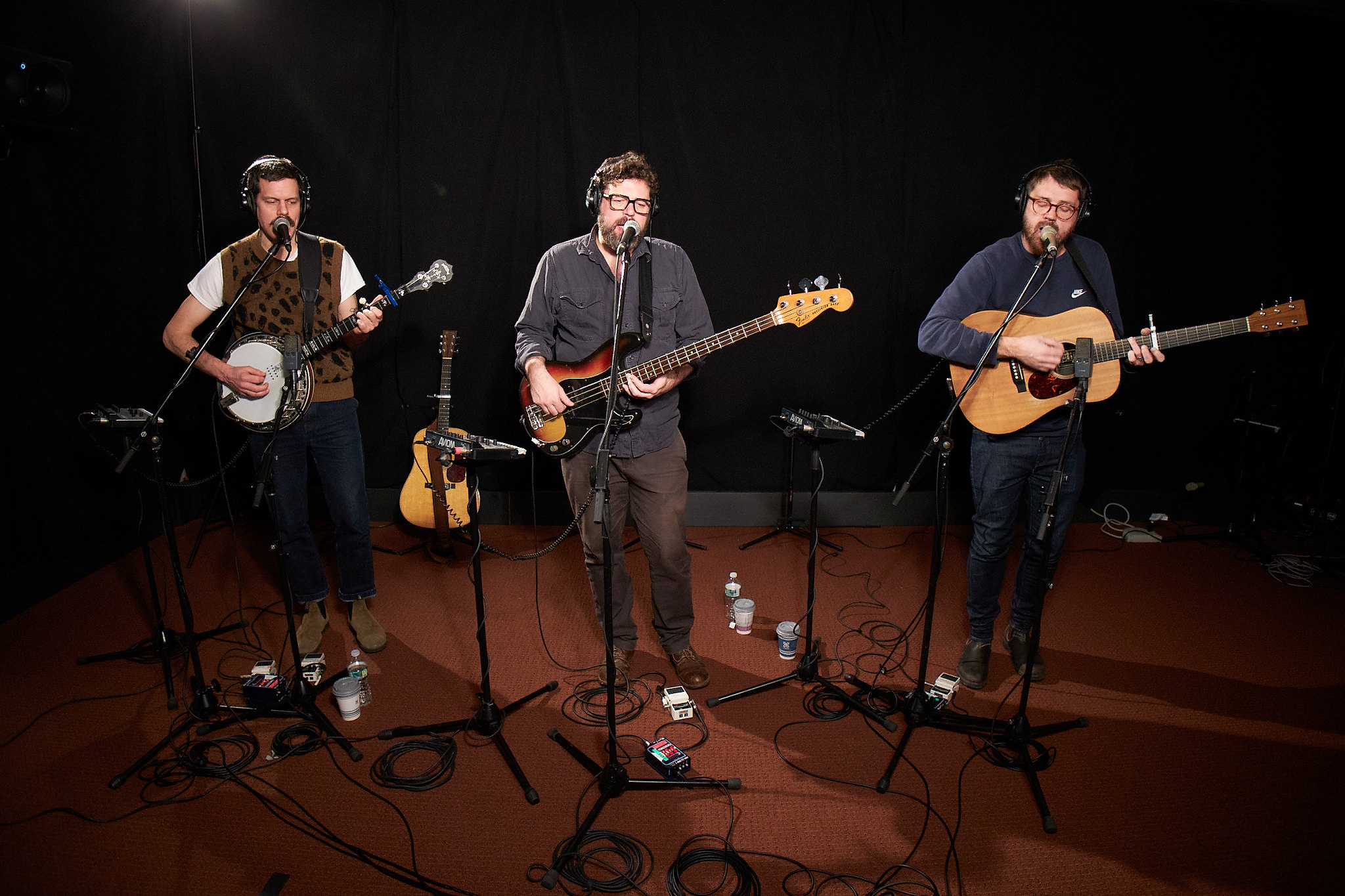This detailed image depicts three musicians in a recording studio engaged in a musical performance. The indoor setting features a maroon or brownish floor with numerous black cords snaking to various microphone stands. 

On the right, a gentleman stands playing an acoustic guitar. He is about six feet tall, with brown hair, a brown beard, and brown glasses. He wears a blue long-sleeve shirt, black shoes, and is positioned behind a microphone stand.

At the center, another gentleman plays an electric guitar. He sports a black shirt, black pants, and brown shoes. His brown hair and beard are partially obscured by black glasses and headphones. He stands behind a microphone that is mounted on a black stand.

On the left, the third musician is playing a banjo. He wears blue jeans and a distinctive leopard-print (or cheetah-print) sweater vest over a white t-shirt. His brown shoes and headphones complete his outfit. He, too, is positioned behind a microphone on a black stand.

All three men are singing into their microphones while playing their respective instruments, contributing to the vibrant musical atmosphere of the studio.